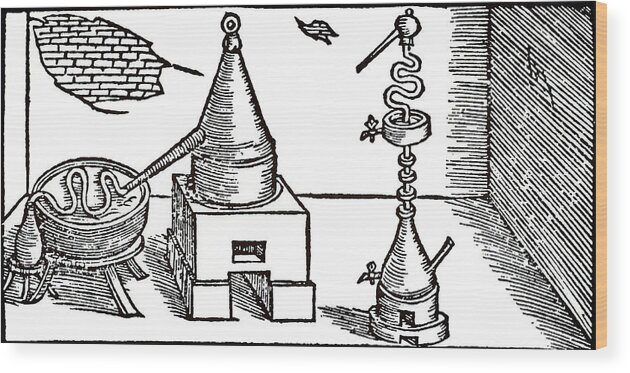This grayscale black-and-white woodcut features a detailed, intricately designed scene of what appears to be an alchemical distillation process set in a dilapidated room. The back wall, with its crumbling plaster revealing bricks underneath, offers a stark contrast to the shaded right-hand corner of the room. On the left side, a jagged break in the wall further emphasizes the room's worn state.

In the foreground, central to the composition, is a complex distillation apparatus. A conical structure, akin to a capital "A," sits prominently on a block. From this central cone, a tube leads into a squiggly pipeline that seems to be encased in a water-filled barrel, ending in a flask perched on a three-legged stool.

To the right, another curious contraption catches attention. This apparatus, reminiscent of a bird with a crane's head or even a fanciful marijuana bong, features a conical top with a convoluted tube and a small bulb with a spout pointing inward. The entire apparatus exudes a sense of archaic, scientific experimentation, capturing both the intricacy of the distillation process and the decaying grandeur of its setting.